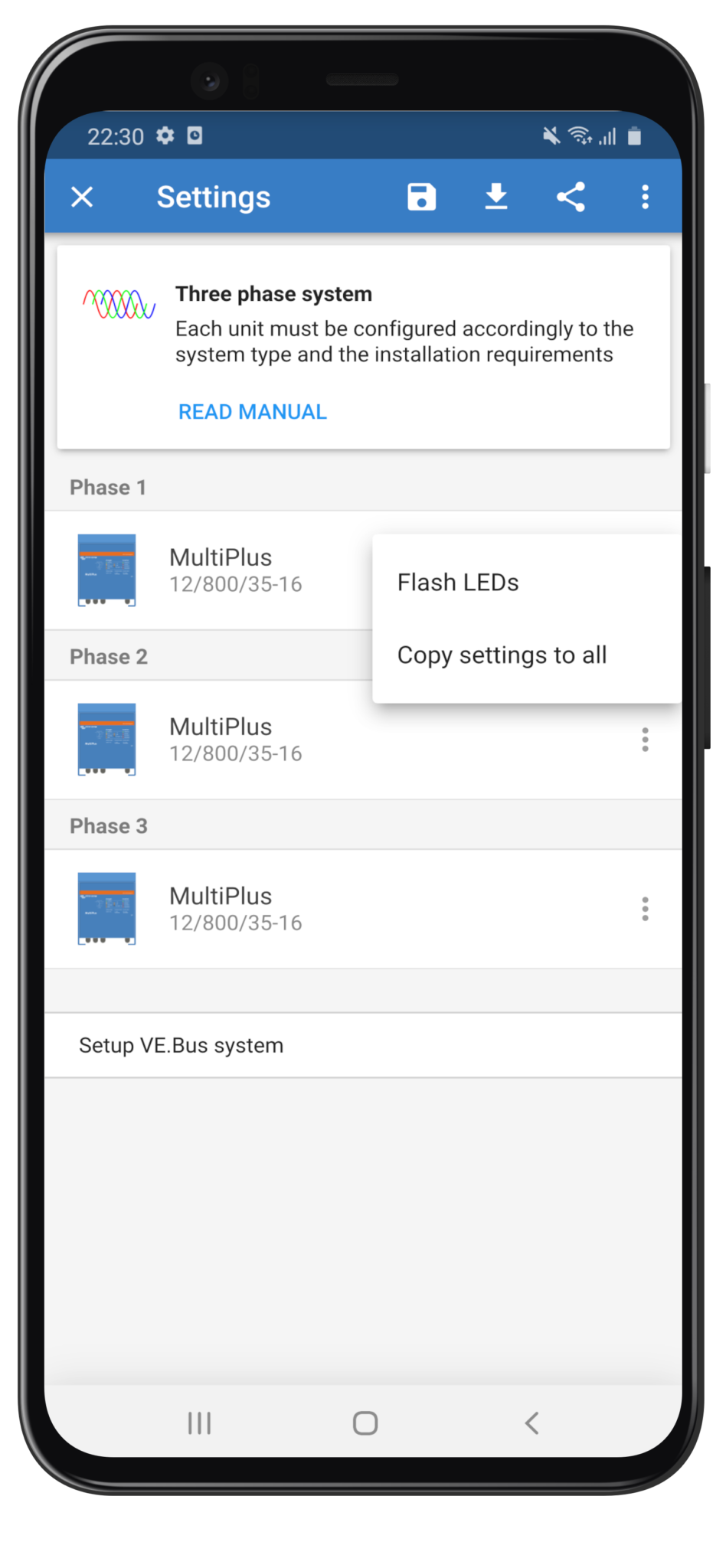The image depicts a smartphone, resembling an iPhone, with its screen prominently displayed. The device features a black frame surrounding the screen, with a black background that gracefully curves around the top edge. At the very top of the screen, there is a dark blue banner displaying the time as 22:30. Adjacent to the time, icons indicate the cell signal strength, an alarm, Wi-Fi signal, and battery level.

Beneath this, a brighter blue banner appears, containing an 'X' on the left side, and the word 'Settings' in white, capitalized print. This banner also includes a downward arrow line, a share icon, and a vertical three-dot menu on the right side.

The main content area features a white background with a centrally positioned square. Within this square, text reads 'Three Phase System,' followed by instructions stating, "Each unit must be configured accordingly to the system type and the installation requirements." Below this, in blue text, the phrase 'Read Manual' is prominently highlighted.

Further down, the screen lists phase configurations:
- Phase One: MultiPlus
- Phase Two: MultiPlus
- Phase Three: MultiPlus

A small pop-up window provides additional options: 'Flash LEDs,' 'Copy Settings to All,' and at the very bottom, a button labeled 'Set Up VE.VUS System.'